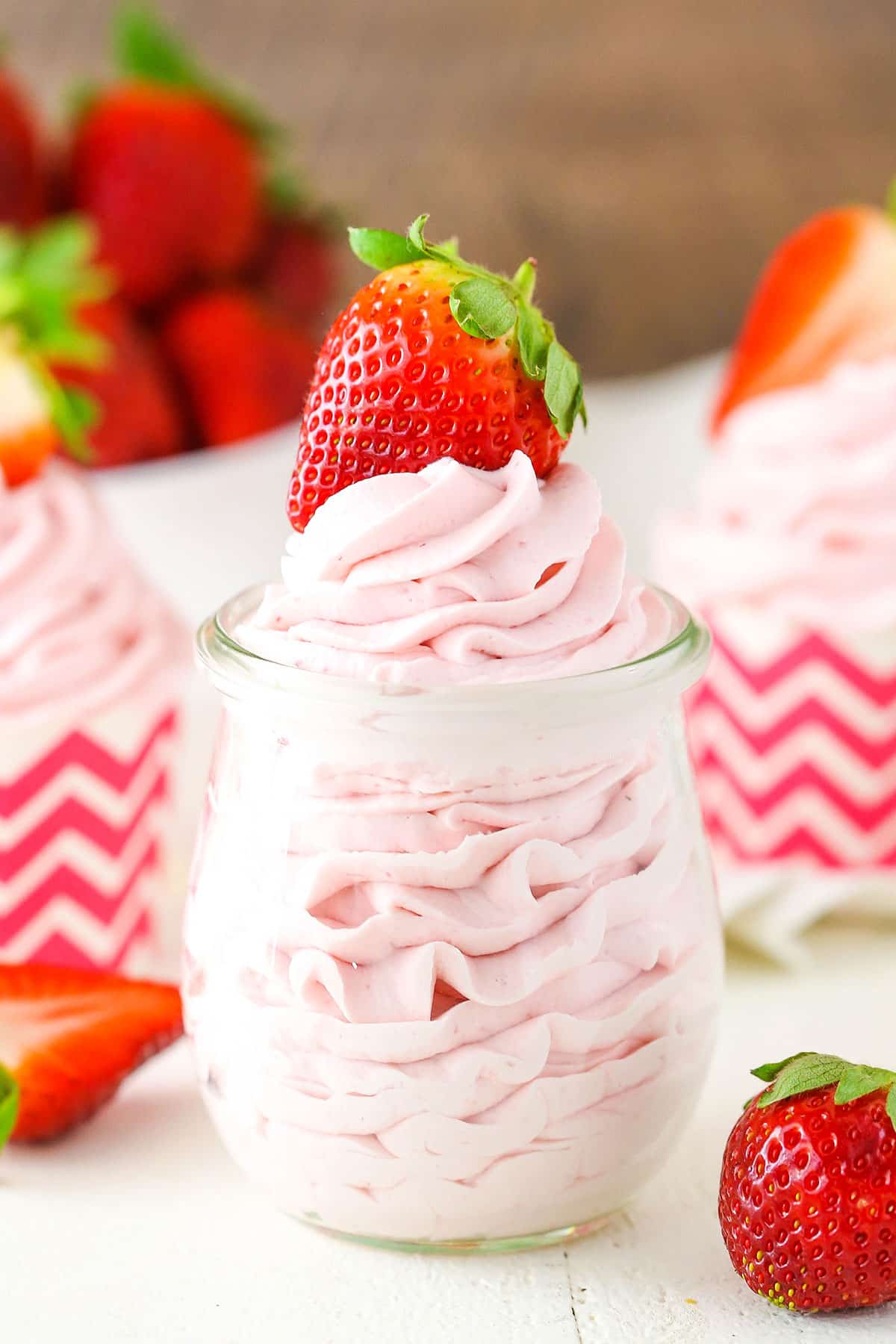This close-up photograph showcases a delectable dessert presented in a clear glass bowl, featuring a generous serving of pink strawberry ice cream, yogurt, or whipped cream that slightly overflows the top. Positioned on the creamy peak is a brilliantly red, ripe strawberry. To the right of the glass on a wooden white table lies another whole strawberry, and to the left sits a strawberry cut in half. The background reveals additional dessert cups adorned with jagged pink and white stripes, also filled with the same pink cream and topped with strawberries. Behind these cups, there is a bowl brimming with vibrant, uncut strawberries, completing the strawberry-themed arrangement. The backdrop displays a brown wall, adding a warm and rustic touch to the scene. The composition is text-free, allowing the vivid colors and textures of the dessert to capture full attention.